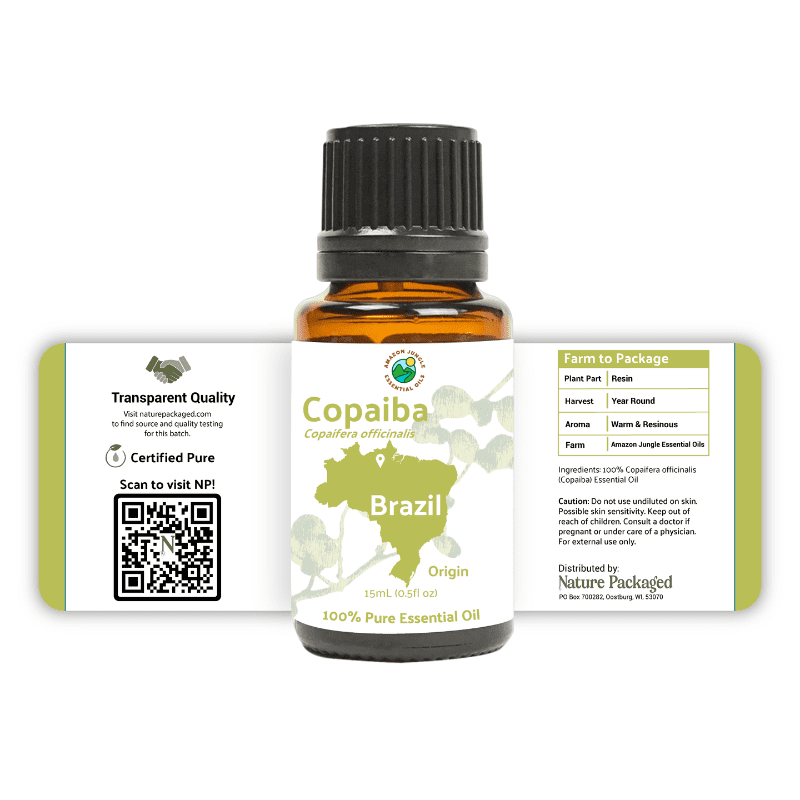The image showcases a small glass vial, approximately a couple of inches tall, containing an orange liquid, which is 100% pure essential oil. The vial, with a brownish hue, is capped with a black lid. The label on the front prominently displays the word "COPAIBA" (C-O-P-A-I-B-A) and includes a silhouette of Brazil in light green with the text "Brazil" inside. Below, it states "origin," "15 milliliters (0.5 fluid ounces)," and "100% pure essential oil." The label extends on both sides for better readability. 

On the left side, the details include a call for "transparent quality," a prompt to visit naturepackage.com for source and quality testing information, certification of purity, and a QR code labeled "scan to visit NP." The right side provides further specifications: "farm to package," "plant part: resin," "harvest: year-round," "aroma: warm and resinous," and "farm: Amazon Jungle Essential Oils." The label is meticulous in its detailing, encompassing both ingredient and caution lists as well as distribution information by "Nature Packaged," set against a clean white background.